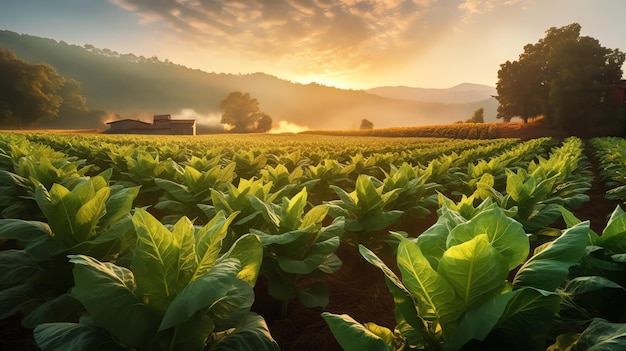This detailed image captures a pastoral scene of a sprawling farm field vividly illustrated or AI-enhanced, possibly blending digital art with a hint of realism. At the forefront, the focus is on verdant heads of lettuce filling the expansive field, meticulously depicted down to the small holes in the dirt where stems emerge. The lush crops stretch out towards the horizon, flanked by green hillsides dotted with trees. In the background, a modest farmhouse or barn stands at a considerable distance, its details softened by the span of the field, yet it's enveloped by a cluster of trees. The scene is set under a pale blue sky, awash with sunlight and punctuated by large, fluffy white clouds. The contrasting hues of deep green plants, darker green trees, and the earthy tones of the distant house create a vivid and serene agricultural tableau.